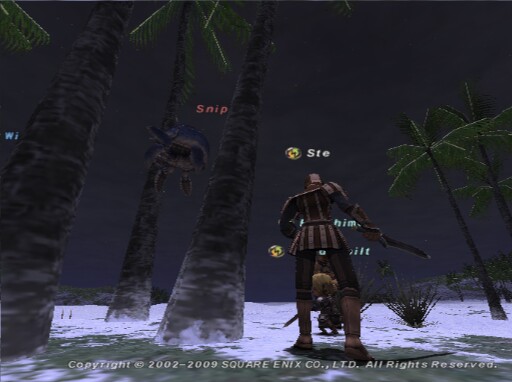This image is a screenshot from a video game, likely taken at night, showcasing a dark black sky with five tall palm trees rising from a sandy area. The sand appears white, with small grassy patches and some plants sticking up from the ground, indicating a low, flat terrain. The perspective is from a low point of view in third person, focusing on a character who is central to the scene. This character wears a tunic and knee-high boots, carrying a weapon, possibly a sword or knife, in his right hand. The character has a blocky head and a striped shirt, evoking a somewhat medieval, non-contemporary attire. Ahead of this character, there is a smaller, barely visible figure also holding a weapon. The image contains a notable red text that reads "snip" between two of the palm trees. At the bottom of the screenshot, there is a copyright notice: "Copyright 2002 to 2009 Square Enix Company LTD, all rights reserved."